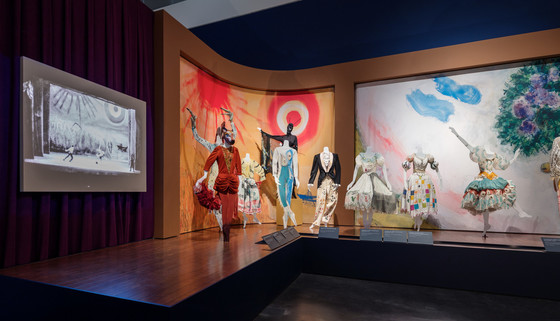The photograph features a museum exhibit displayed on an L-shaped wooden shelf. The exhibit showcases a variety of vibrant, vintage costumes worn for a musical or play, all meticulously arranged on mannequins. The clothing includes an array of styles and colors, such as a red billowy pants and blue bodysuit, a black suit with flowy white floral pants, a white dress, and other dresses. Behind the mannequins, large, curved murals of artwork with Japanese or Chinese origins add a colorful backdrop. Additionally, there is a large screen on the left side of the image that shows a black and white photo, possibly depicting the original wearers of these costumes, adding a historical context to the display.